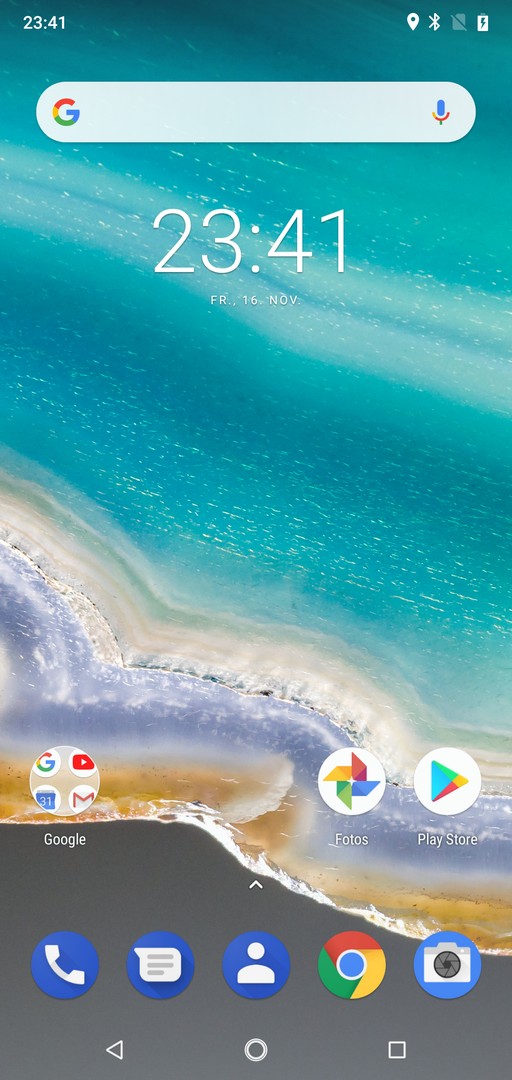The image depicts a screenshot of a cellphone’s home screen. Prominently, at the center, there is an oval icon featuring Google's recognizable "G" logo along with a microphone symbol, indicating voice search functionality. Directly beneath this icon, the time is displayed in bold white numbers, "23:41". Below the time, in much smaller white text, the date is noted as "Friday the 16th, November".

The background of the screen showcases a serene water scene, transitioning from light blue, resembling shallow waters near the edge of sandy terrain, to a darker blue, indicative of deeper waters. This background hints at an aerial perspective of a coastal area.

At the bottom part of the screen, lined up within the dock, there are various app icons. First is the Google folder, containing multiple Google app icons within a circle. Adjacent to this, there are individual app icons including "Photos", represented by a windmill-like emblem of colorful petals, and the "Play Store", symbolized by a triangular icon interspersed with colors.

Additionally, on the home screen, there are several circular app icons: A white telephone handset symbol inside a blue circle for making calls; a blue circle containing a piece of paper, likely representing a document or notes app; another blue circle, this time with a little man icon, signifying a contacts or people app; a multicolored circular icon with segments of red, yellow, and green surrounding a central blue circle with white outlining, probably representing Google Chrome; and lastly, a blue circle with a camera emblem, indicating a camera or photos-related application.